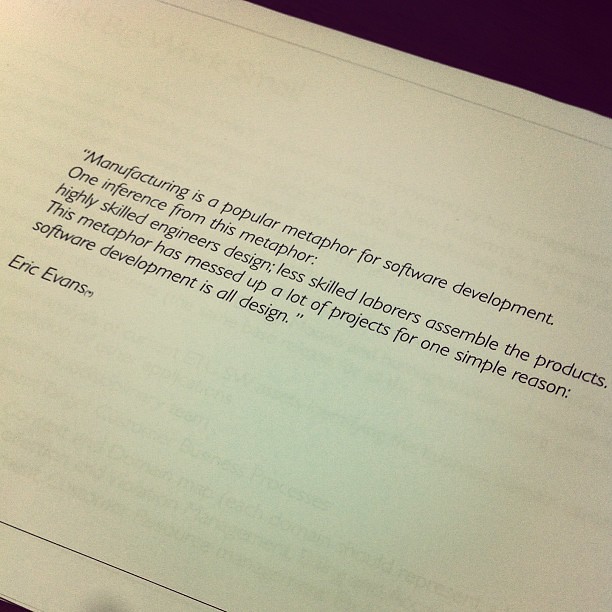The image showcases an ivory-colored sheet of paper with black text, partially cut off on the top, bottom, and sides. Positioned against a black background, the paper is tilted slightly to the right. The text reads: "Manufacturing is a popular metaphor for software development. One inference from this metaphor, highly skilled engineers design, less skilled laborers assemble the products. This metaphor has messed up a lot of projects for one simple reason. Software development is all design." Below this quote, the name "Eric Evans" appears in black letters. The writing is printed in a basic, conventional font, and there are traces of faded writing beneath and around the primary text. The overall scene is tinged with a dim yellowish glow, suggesting low lighting, and the page appears to be part of an open book laid flat on a wooden table.